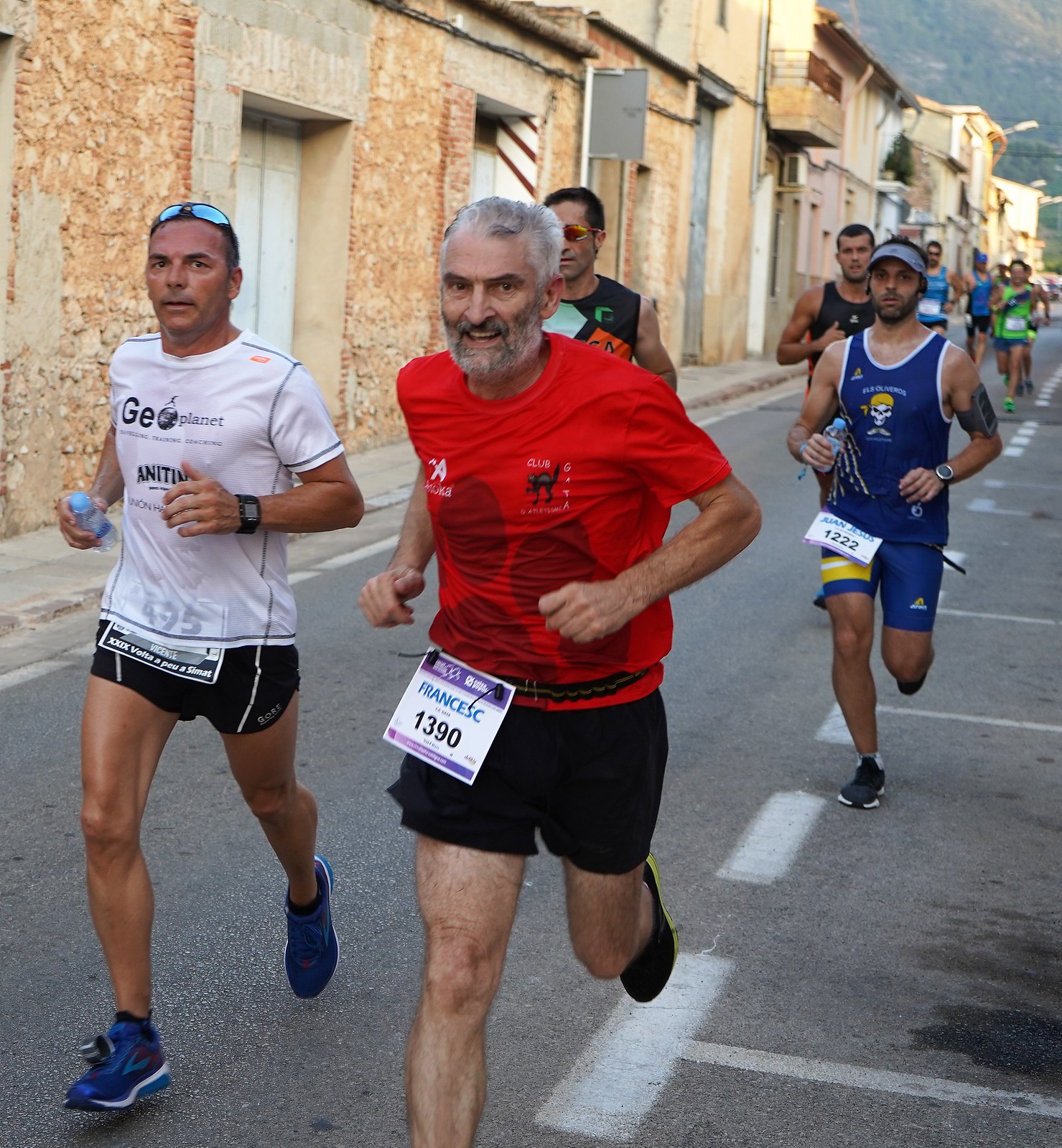The photograph captures a lively race taking place on the narrow, single-lane streets of a small city or town. Approximately 20 to 30 runners, mostly men, are moving towards the camera on a paved road marked with gray lines and a dotted white centerline. The runner in the forefront sports a red short-sleeve shirt, black shorts, and black shoes with a yellow stripe. He has gray hair and a beard, and his race number is prominently displayed as "1390" on a white and purple sign. Beside him, a runner in black shorts and a white t-shirt with the number "495" stands out, wearing blue tennis shoes, and sporting sunglasses on his head, and a watch on his arm. The background reveals picturesque, closely-knit old stone buildings typical of small cities, juxtaposed against a distant, majestic mountain. Other runners, arrayed in varied outfits—blue tank tops, visors, and colorful t-shirts—continue to fill the scene, emphasizing the communal and vibrant spirit of the race.